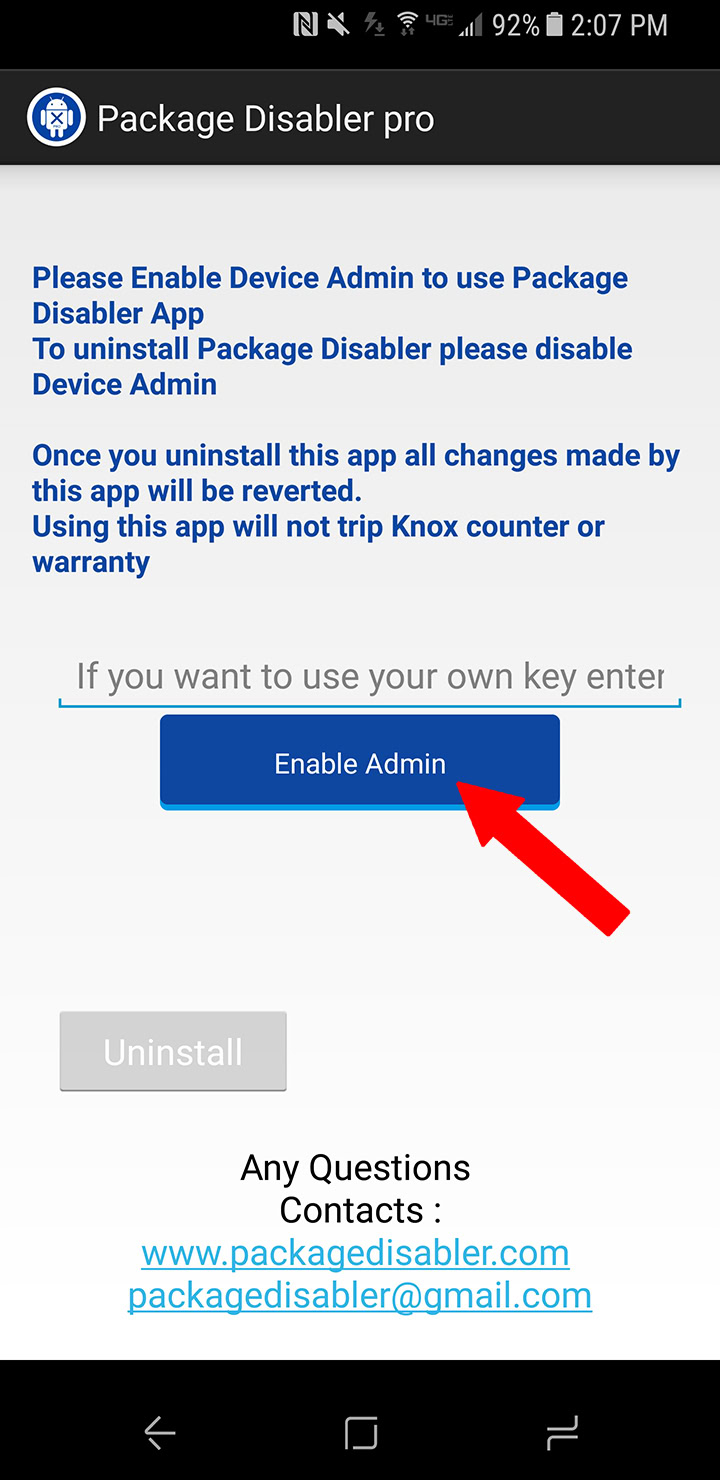### Detailed Caption:

The screenshot depicts a mobile device interface with a white background, taken at 12:07 p.m. with the battery level at 92%. The central focus of the screen is a black rectangular notification from the "Package Disabler Pro" app. Nestled within the notification is a blue circle featuring a white robot icon. Next to it, in blue text, a prompt reads: "Please enable device admin to use Package Disabler. Apps to uninstall Package Disabler, please disable device admin. Once you uninstall this app, all changes made by this app will be reverted. Using this app will not trip Knox counter or warranty."

Beneath the main text is a blue line, followed by a black text field that says: "If you want to use your own key, enter it here." Adjacent to this text field is a blue rectangle labeled "Enable Admin" in white text, highlighted with a red arrow pointing towards it. Below this section, a gray rectangle reads: "Uninstall" in white text.

In case of any questions, the message suggests contacting the support team, offering two email addresses in blue: "www.packagedisabler.com" and "packagedisabler@gmail.com." Lastly, at the bottom of the screenshot, there is a black rectangle with a left arrow icon, likely indicating a navigation option.